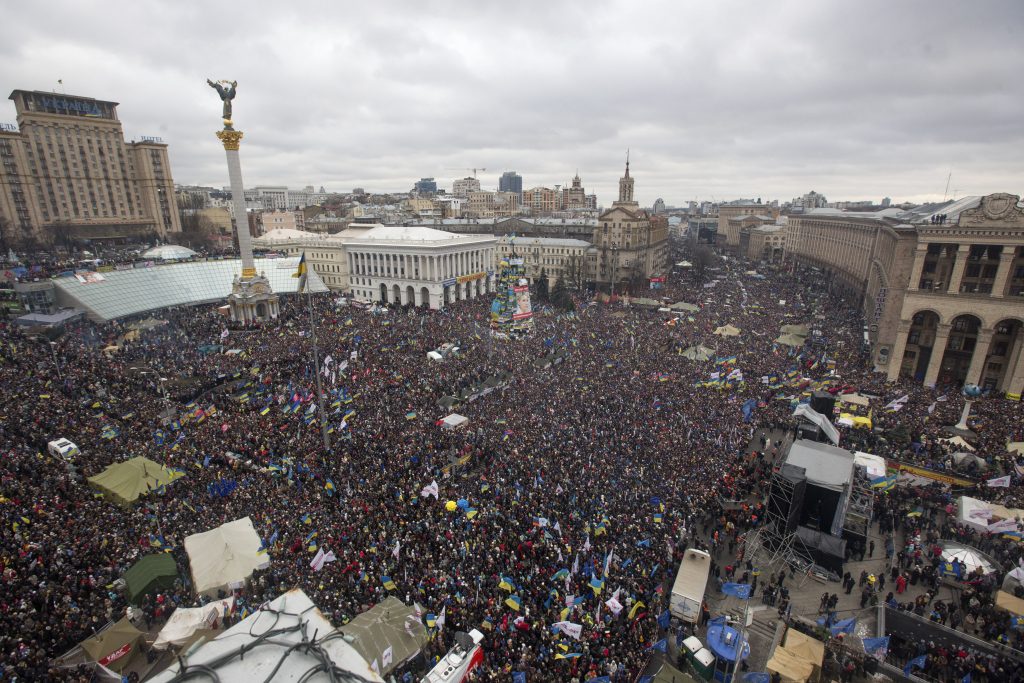This aerial view captures a massive crowd assembled in a city for what appears to be a significant political rally or global cause. The scene is bustling with hordes of people, resembling a sea of ants from this height. The sky is overcast with gray clouds, adding to the somber atmosphere. Among the urban sprawl, a mix of low and tall buildings can be seen. Central to the image is a tall, white column topped with a statue, which stands on an imposing pedestal resembling a building. The crowd is densely packed around a small square located near the bottom left of the middle of the image. To the upper left and middle right, large beige buildings are notably visible. On the right bottom corner, there's a less populated area with some scaffolding and a white 18-wheeler truck. Military-type tents are scattered around, indicating the gravity of the event. A subtle hint suggesting the location might be Ukraine is visible through a Ukrainian flag. It’s a powerful image of social gathering against a backdrop of architectural grandeur and a cloudy sky.